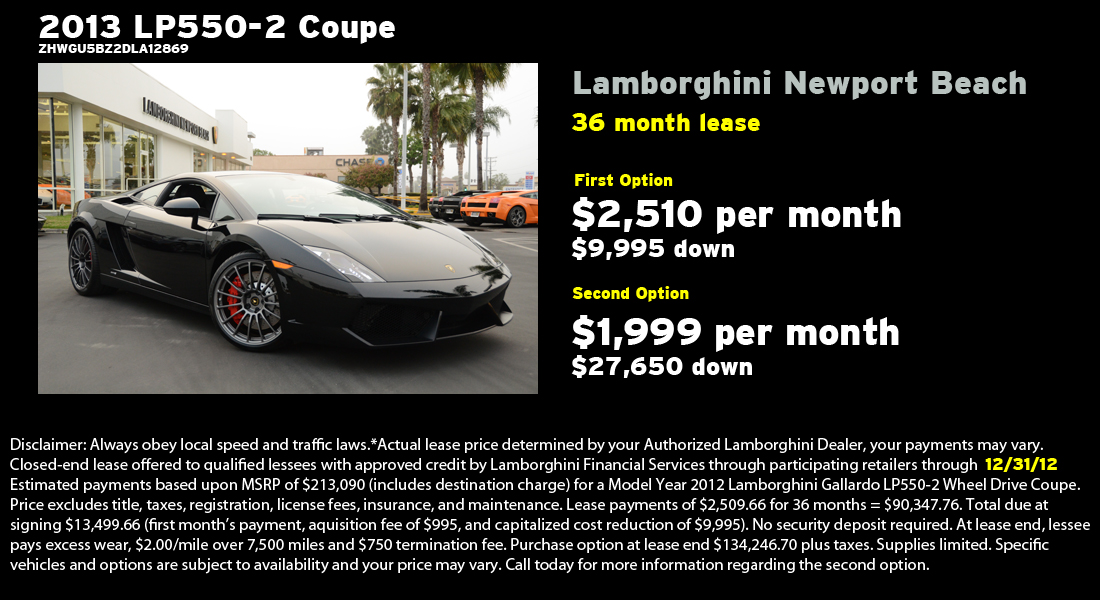This image is a detailed sales ad for a 2013 Lamborghini LP550-2 Coupe, set against a black background. On the left side, a photo showcases the sleek black sports car parked in a Lamborghini dealership lot, characterized by palm trees and an overcast sky. The car features striking aluminum mag rims and red brake calipers, embodying a powerful and luxurious design.

Above the car’s image, bold white text announces "2013 LP550-2 Coupe", followed by the vehicle's VIN "ZHWGU5BZ2DLA12869". Adjacent to this, the dealership name "Lamborghini Newport Beach" is displayed in gray font.

Two leasing options are prominently featured. The first option, highlighted in white, offers a 36-month lease at $2,510 per month with $9,995 down. The second option, in yellow, advertises a lease at $1,999 per month with a higher down payment of $27,650.

A comprehensive white text disclaimer at the bottom informs potential buyers of lease terms, including a closed-end lease, qualification conditions, specific financial details such as MSRP, associated due amounts at signing, and additional fees. The disclaimer also mentions the lessee's responsibilities, options at lease end, and emphasizes compliance with local speed and traffic laws.

Overall, this ad combines visual and textual elements to provide extensive information about leasing a high-end Lamborghini vehicle, enticing potential customers with its detailed presentation and financial offerings.